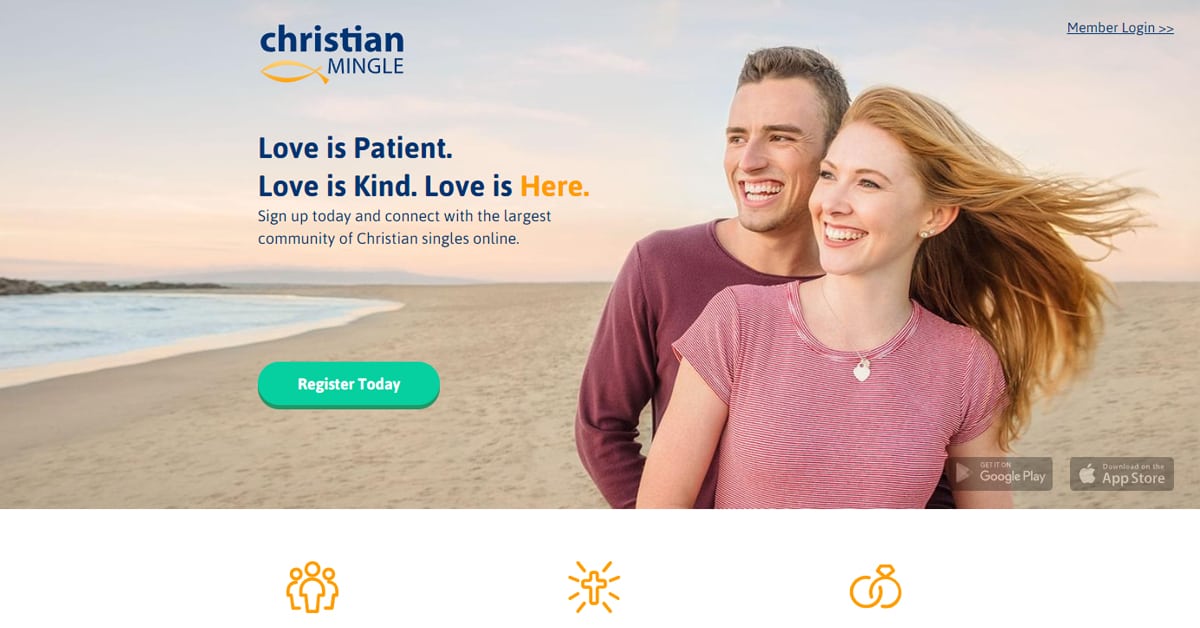This screenshot captures the homepage of a dating site called Christian Mingle in a banner style. Dominating the top of the page is a large banner featuring a white man and a white woman on a beach, both smiling and gazing thoughtfully into the distance, where a lake is visible. The banner prominently displays the Christian Mingle logo accompanied by the phrase "Love is patient. Love is kind. Love is here." The word "here" is highlighted in yellow text, contrasting with the blue text of the rest of the sentence. Below this, a call to action reads: "Sign up today and connect with the largest community of Christian singles online."

A green button labeled "Register Today" stands out in the bottom-right corner of the banner. Additional options to download the Christian Mingle app are provided via two buttons corresponding to the Google Play Store and the Apple App Store. A member login link is subtly positioned in the upper right-hand corner. 

Beneath the banner, there are three yellow icons on a white background: one of a group of people, one of a cross, and one representing marriage with two interlocking rings. These icons succinctly represent the community, faith, and relationship focus of the site.